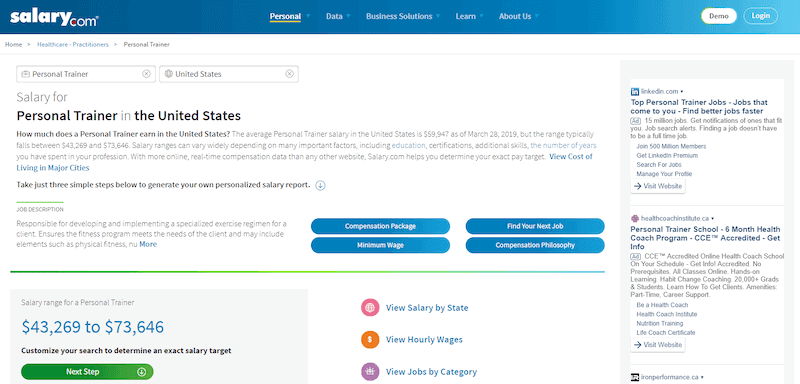The image displays the homepage of the website Salary.com. At the top of the page, there is a gradient banner that transitions from a darker blue on the left to a bright light blue on the right. On the left side of the banner, the text "salary.com" is prominently displayed. The word "salary" is in bold, lowercase, white letters, while the period is marked by a red dot, and "com" is in a finer white print.

Moving to the right, several menu options are listed horizontally, each accompanied by a drop-down menu. These options include "Personal," which has a yellow underline, "Data," "Business Solutions," "Learn," and "About Us." Beside these, there are buttons for "Demo" with a white background and "Log In" with white text.

Below the navigation bar, there are options like "Home," "Healthcare Practitioners," and "Personal Trainer." Further down, the page focuses on a detailed description of a personal trainer's salary in the United States. The text reads, "Personal Trainer, United States - Salary for a personal trainer in the United States. How much does a personal trainer earn in the United States?" Following this inquiry, a short description is provided.

The page also invites users to take "just three simple steps to generate your own personalized salary report" and includes a section labeled "Job Description." Below this, a green line delineates the salary range for a personal trainer, which is stated as $43,269 to $73,646, and offers an option to "Customize your search to determine an exact salary target." At the bottom of this section, a green banner with the text "Next Step" in white encourages further action.